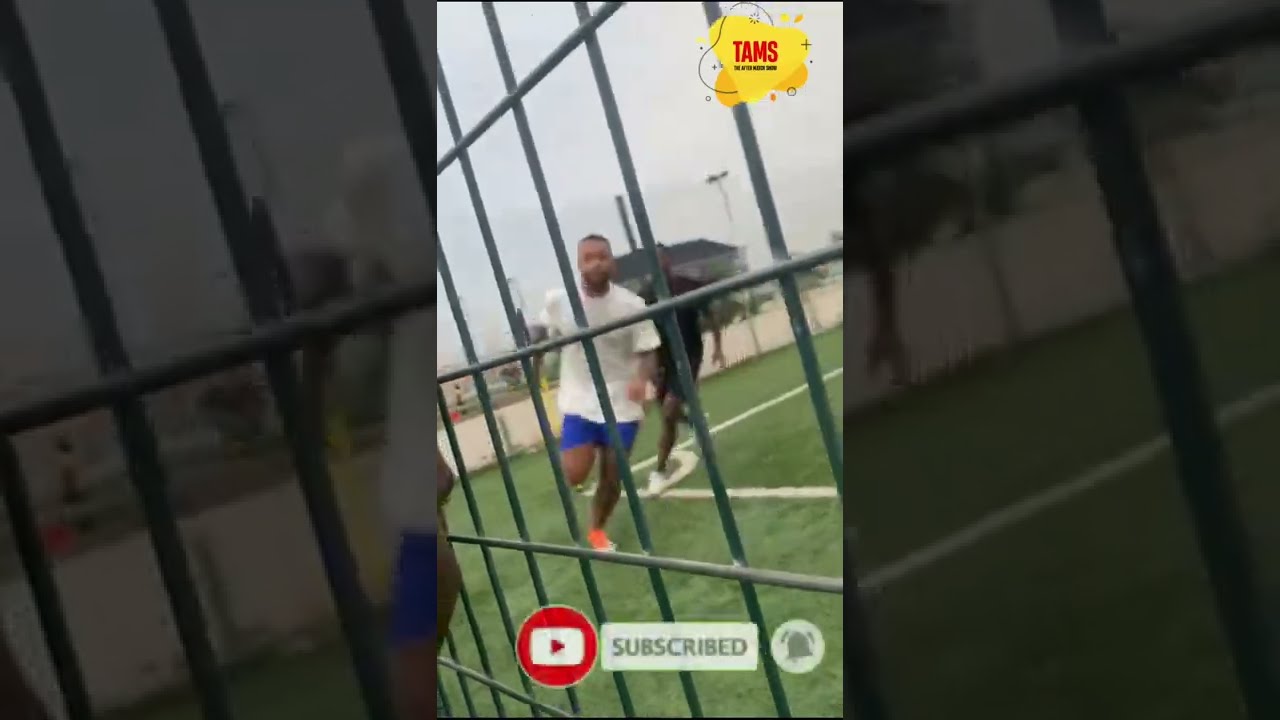The photograph captures a dynamic moment of two men running on a field enclosed by a greenish-gray fence. The focal point is a man in a white t-shirt, blue shorts, and orange sneakers, running towards the camera, with the image slightly blurred. Another man in black attire follows closely behind him, near a visual marker resembling a baseball base. The background displays a tall white wall and a gray building. The image is divided into three sections: the central view and two semi-transparent close-up views on either side. Additionally, a YouTube play button, a "Subscribed" label, and a notification bell icon are visible at the bottom of the image, suggesting a screenshot from a video. The green field beneath the runners shows lines reminiscent of a baseball diamond, although there is no specific soil path visible.